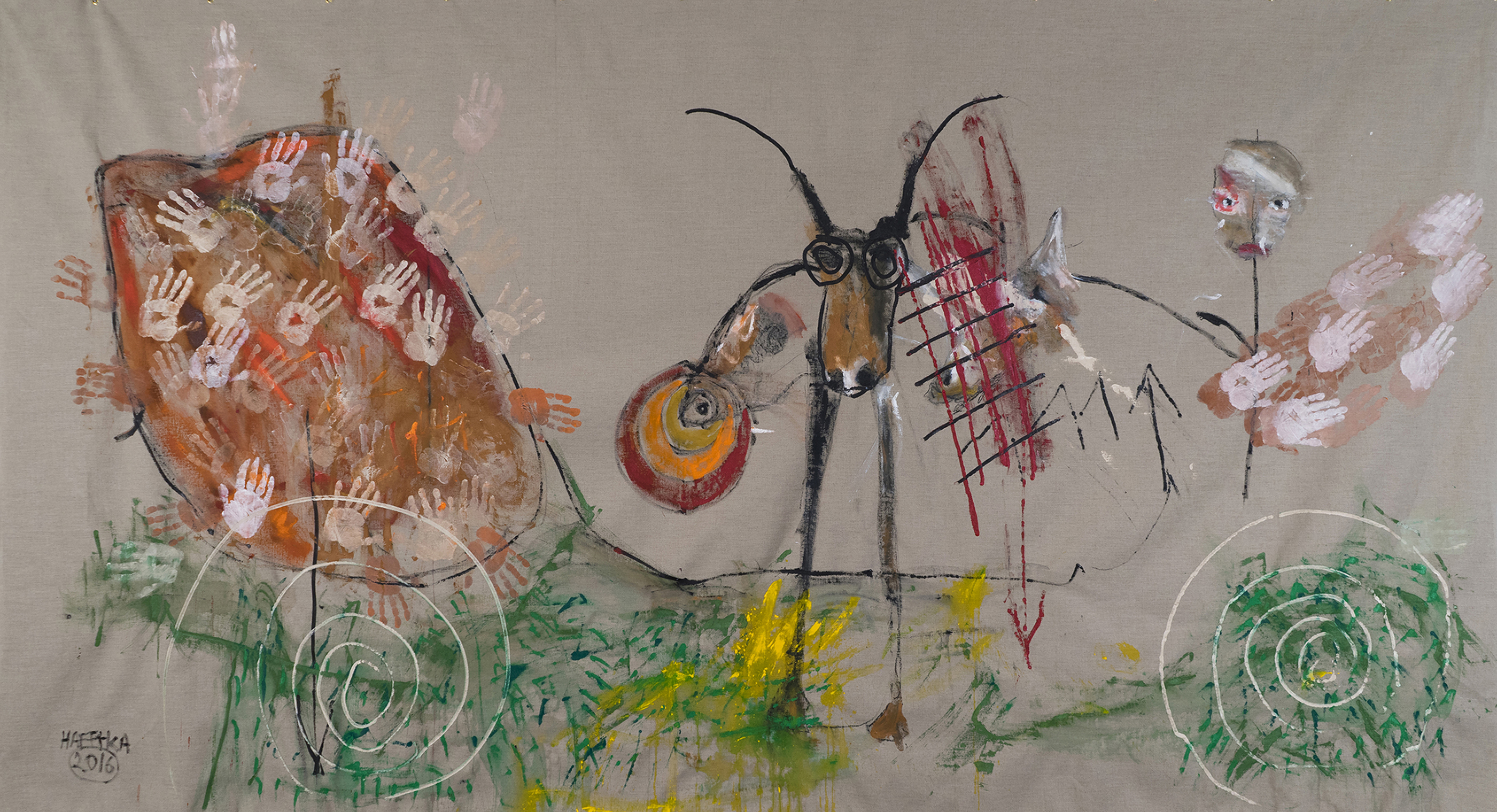This painting, titled "Bicameral Mind" by Michael Haftka and created in 2016, is a striking example of figurative expressionism with its abstract and surreal elements. The landscape-oriented, narrow horizontal format captures the viewer’s attention with an intricate blend of colors and forms. 

On the left side, a notable feature is the abundance of white handprints irregularly covering a brown, rock-like shape. These handprints, approximately 40 or more, create a chaotic yet compelling texture. Surrounding the handprints are blotches of yellow and green, enhancing the abstract feel of the painting.

In the center, the main subject is a bizarre stick figure with a deer-like head adorned with antlers and spectacles, which gives it a uniquely quirky appearance. The figure stands on two long, slender legs devoid of a body, adding to the surreal nature. Its left arm features more white handprints, particularly around the shoulder. In its right hand, it holds a round, orange and red circular object, possibly representing a ball.

To the right of this central figure is an unsettling face with two eyes, no nose, and lips, painted atop what resembles a flower stem, contributing to the dreamlike quality of the scene. Additional handprints, along with the splashes of colors such as red, green, and yellow, further enrich the complex, multi-layered composition.

Overall, the painting communicates a sense of whimsical and eerie abstraction, inviting viewers to delve into its myriad of details and interpret its enigmatic themes.